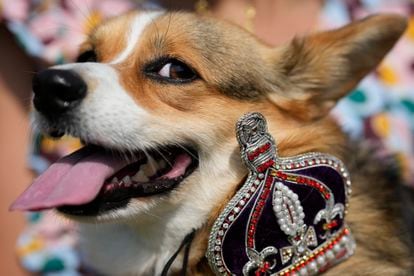The image is a high-resolution photograph of a small Welsh Corgi dog with brown and white fur. The dog's head is pointed to the left but slightly tilted back toward the right, giving the appearance of a panting smile. Its ears are perked up, and it is glancing sideways to the right of the image with a side-eye expression. The Corgi is adorned with a decorative crown located near its shoulder; the crown features black and metallic silver colors with pearls at the base and center, and red embellishments. The background of the image is blurred, hinting at possible decorations, which suggests the photo might have been taken at a pet celebration or competition. There is also an indistinct figure visible behind the dog, adding depth to the scene.